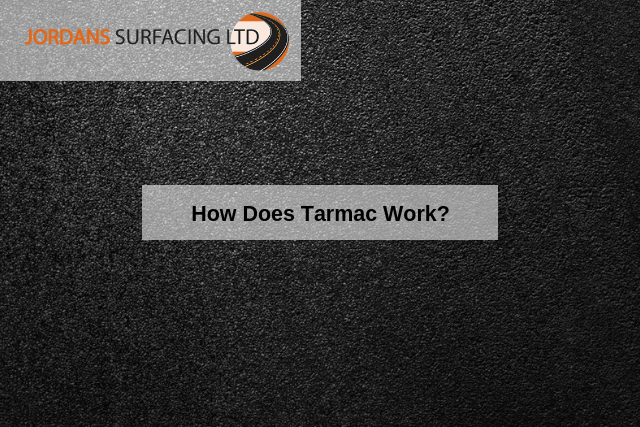The image is a rectangular, black, textured background that is wider than it is tall, possibly part of a sales presentation by a resurfacing company. In the upper left corner, there is a light gray rectangular area containing the company name "Jordan's Surfacing Ltd" in orange and black text. This section is partially overlaid with a logo that depicts a black highway with orange stripes and a white outline. Centered in the middle of the image is a gray oblong box with black text that reads, "How Does Tarmac Work?" followed by a question mark. The overall aesthetic of the image suggests a professional, minimalist design with a focus on information and branding.